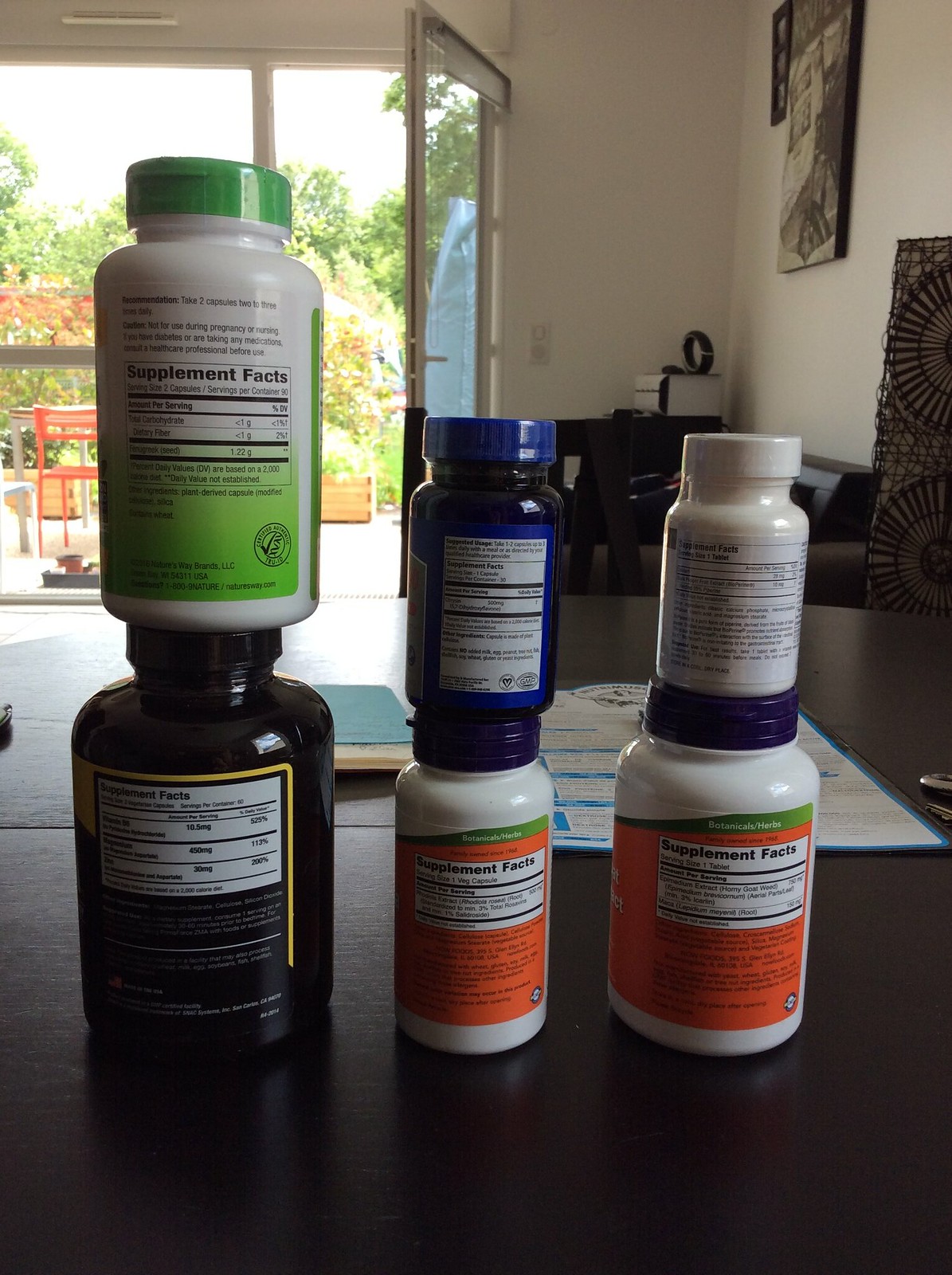The photo depicts six bottles of supplements arranged in a visually organized manner on a dark wooden table. The bottles are displayed in two vertical columns, with three bottles in each column. The labels are facing outward, showing the "Supplement Facts" section, but the brands and specific contents remain indiscernible due to the small print.

In the left column, the bottom bottle is made of dark plastic with a label featuring a yellow outline around the "Supplement Facts" section. Stacked above it is a white plastic bottle with a green lid and similar labeling. The middle column's bottom bottle is white, featuring a blue lid and an orange label with comparable labeling details. Above it, there is a dark plastic bottle with a blue lid and a blue label. The right column parallels the middle column, with a similar but larger white bottle with an orange label on the bottom and a smaller white bottle with a white lid on top.

The setting is indoors, featuring a backdrop with an open glass door revealing an outdoor area with lush green trees, a red chair, and a brown table. The indoor scene includes a book, some paper, and a set of keys partially visible on the table, along with a chair and a speaker in the background. A frame hangs on the right side wall. The atmosphere suggests a clear, sunny day, enhancing the overall brightness of the scene.